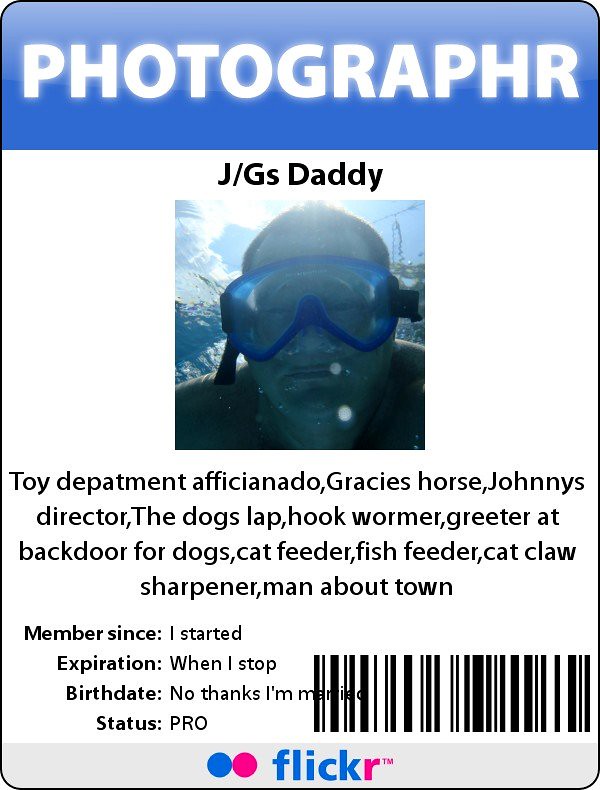This image appears to be a digitally created, vertically oriented identification badge with a playful and whimsical design. The background is predominantly white with various colored elements. At the top, there's a blue header with white all-caps letters that read "PHOTOGRAPHER." Below this, in a white section, it says "J/G's Daddy" in capital letters. Dominating the center of the image is a picture of a man wearing blue goggles, submerged underwater, with sunlight filtering through the water's surface.

Beneath the image, there's text listing a range of humorous titles and roles associated with the person, such as "Toy Department Aficionado," "Gracie's Horse," "Johnny's Director," "The Dog's Lap," "Hook Warmer," "Greeter at Back Door for Dogs," "Cat Feeder," "Fish Feeder," "Cat Claw Sharpener," and "Man About Town." There’s also a barcode located on the right side of the image. At the bottom, there's a light gray banner featuring a blue and pink dot in the center, followed by the word "Flickr" with a trademark symbol. The image incorporates a color palette of blue, white, black, light blue, gray, purple, and pink.